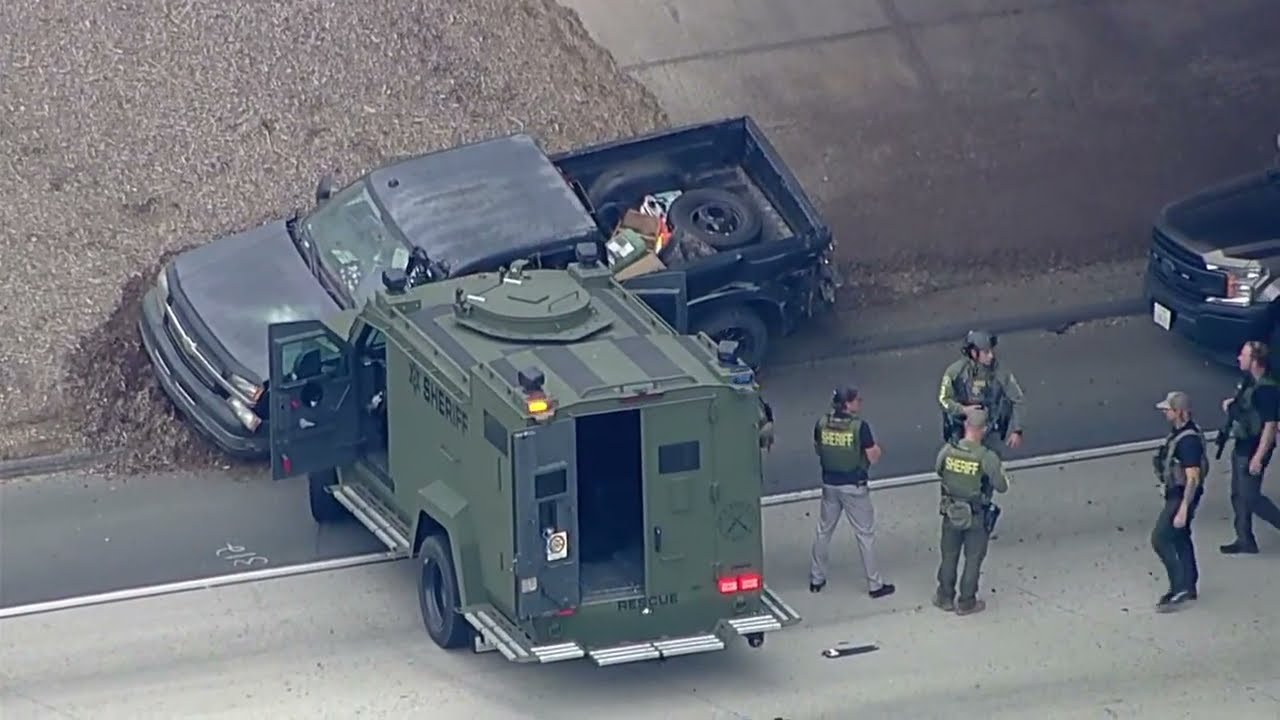This aerial photo, potentially from the roof of a building or drone, captures an intense scene on the side of a major road or freeway. A sheriff's armored truck, in an army green color, has collided with and rammed a black Chevrolet pickup truck, which is now tilted and heavily damaged, particularly at the rear. The pickup truck, laden with debris and a tire in its bed, rests on the dirt shoulder of the road. The driver's and rear doors of the armored sheriff truck are flung open. Surrounding the vehicles are at least five sheriff deputies, identifiable by their green bulletproof vests marked with "sheriff" in yellow letters. Among them is one female officer, and several deputies are equipped with long guns pointed down. One deputy wears a helmet. They appear to be either debriefing or securing the scene. A saw or weapon lies on the ground near them. The detailed nature of the image lends a sense of uncertainty as to whether it is a real-life capture or a highly realistic scene from a video game.